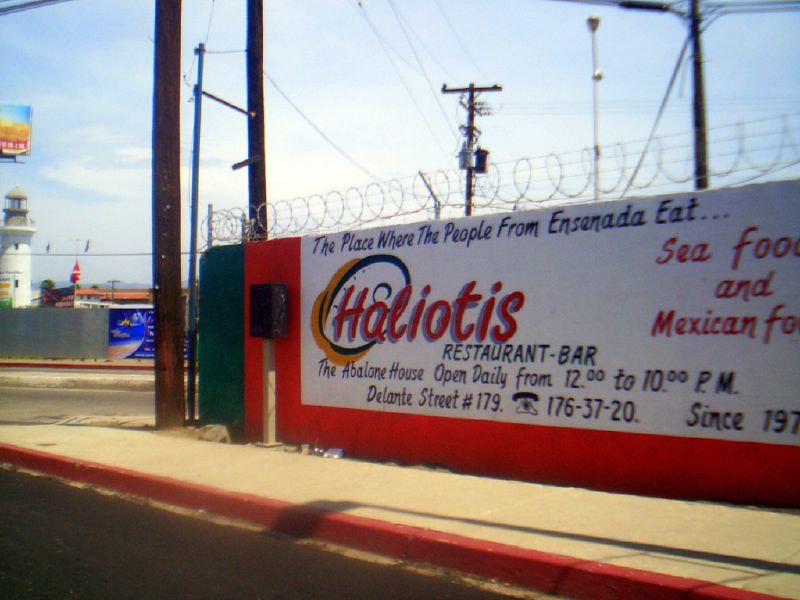The image features a prominent, large, white and red sign situated atop a tan curb with a red edge. The sign is slightly angled to the back left. Behind the sign, there are power lines and utility poles, as well as a grayish-blue fence or wall to the right. In the background, an orange building with a white tower is visible, along with a partially seen advertisement board above the tower.

The sign itself is detailed with various texts. At the top in white writing, it states, "The place where people from Ensenada eat." Below it, in red letters, is the name "Haleoti's Restaurant Bar," although another section mentions it as "Cheliotis," with a distinct blue and yellow "C." Further down, it reads "Restaurant Bar and the Abalone House" in white writing, specifying, "Open daily from 12 to 10 p.m.," and it includes an address, "Delonte Street number 179," as well as a telephone number, "176-3720." The sign also notes "Seafood and Mexican Food," though parts of these words are partially cut off in the image.